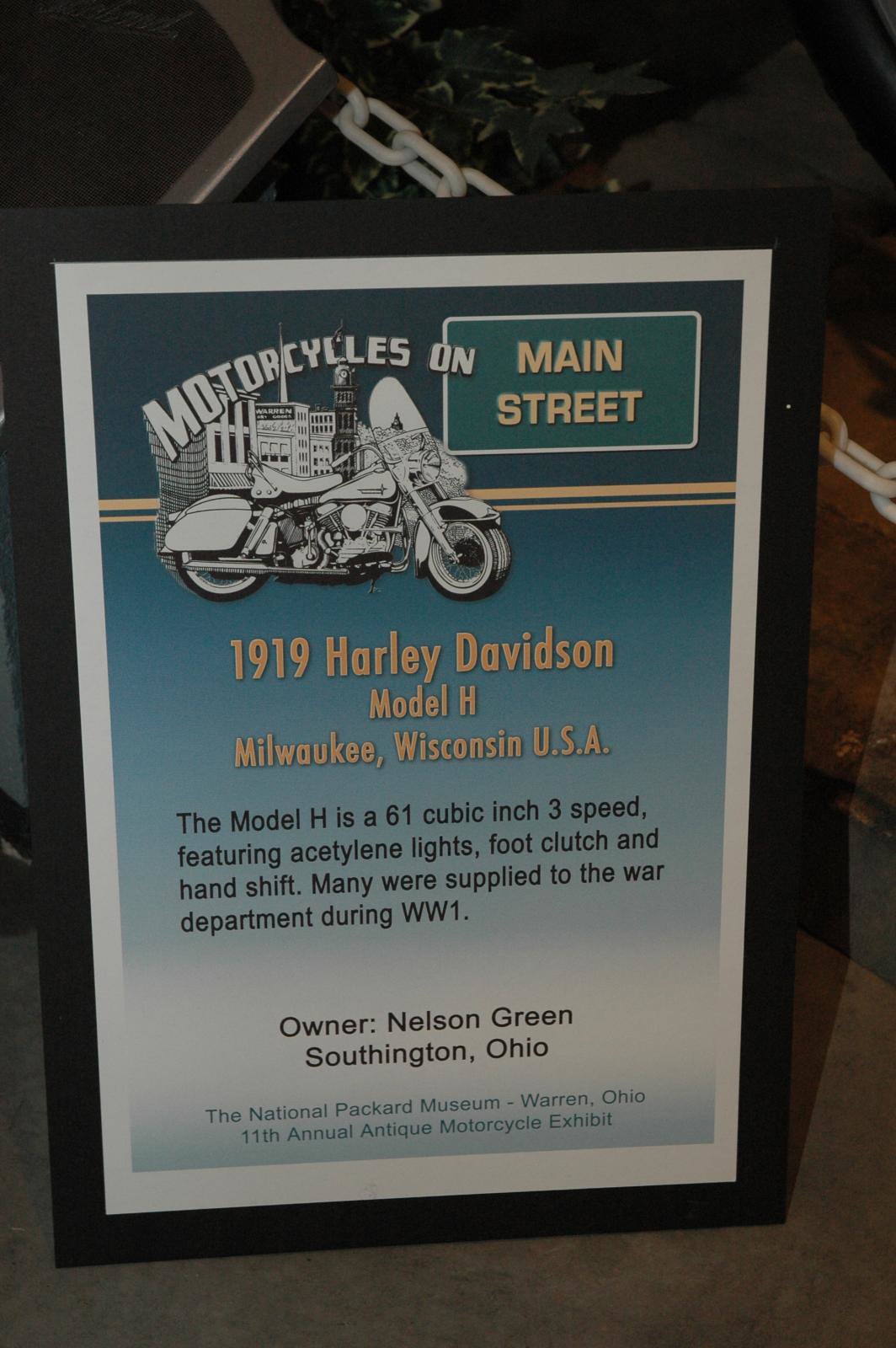The image depicts an informational plaque resting casually against a white chain hanging from a silver metal part. The plaque features a narrow black border followed by a white border, with the background fading from dark blue at the top to white at the bottom. Centered at the top, there’s a black and white illustration of a motorcycle in front of buildings. The top text reads "motorcycles on" in white, followed by a green rectangular box in the upper right corner with yellow lettering that says "Main Street." Below this, in gold text, it states "1919 Harley-Davidson Model H, Milwaukee, Wisconsin USA." Further down, in black text, it describes the Model H as a "61 cubic inch 3-speed featuring acetylene lights, foot clutch, and hand shift. Many were supplied to the War Department during WW1." It also notes the owner as "Nelson Green, Southington, Ohio," and at the very bottom, in blue text, it mentions "The National Packard Museum, Warren, Ohio, 11th Annual Antique Motorcycle Exhibit." The image seems to have been taken casually by a bystander, with chains and the ground visible behind the sign. The plaque is colorful, featuring black, white, green, yellow, and various shades of blue.